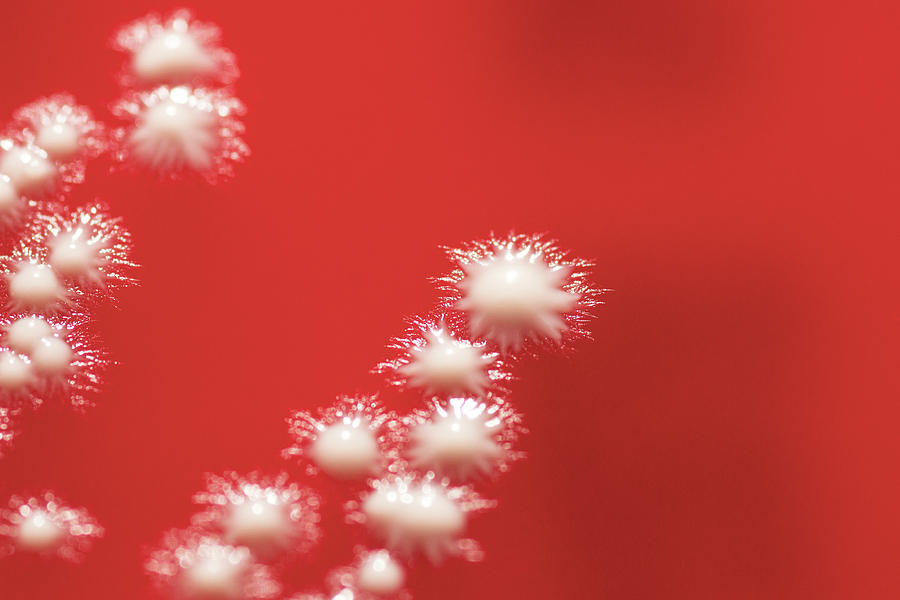The image is a highly magnified microscopic slide with a vividly intense red background, resembling a deep blood red hue. The coloration varies slightly, with darker red tones at the top and bottom edges. Dominating the left and center portions of the image are several clusters of white, circular formations resembling fungal yeast. These waxy-looking clusters, presenting a raised texture, are surrounded by intricate, almost crystalline, striations that branch out like tiny filaments or whiskers. The white formations have multiple fibrous extensions projecting in all directions, creating an intricate, complex pattern. The largest cluster is centrally located, with two additional noteworthy clusters on the left, while the right side of the image remains devoid of any structures. The overall style evokes scientific microscopic slide photography, capturing detailed and precise fungal yeast formations.